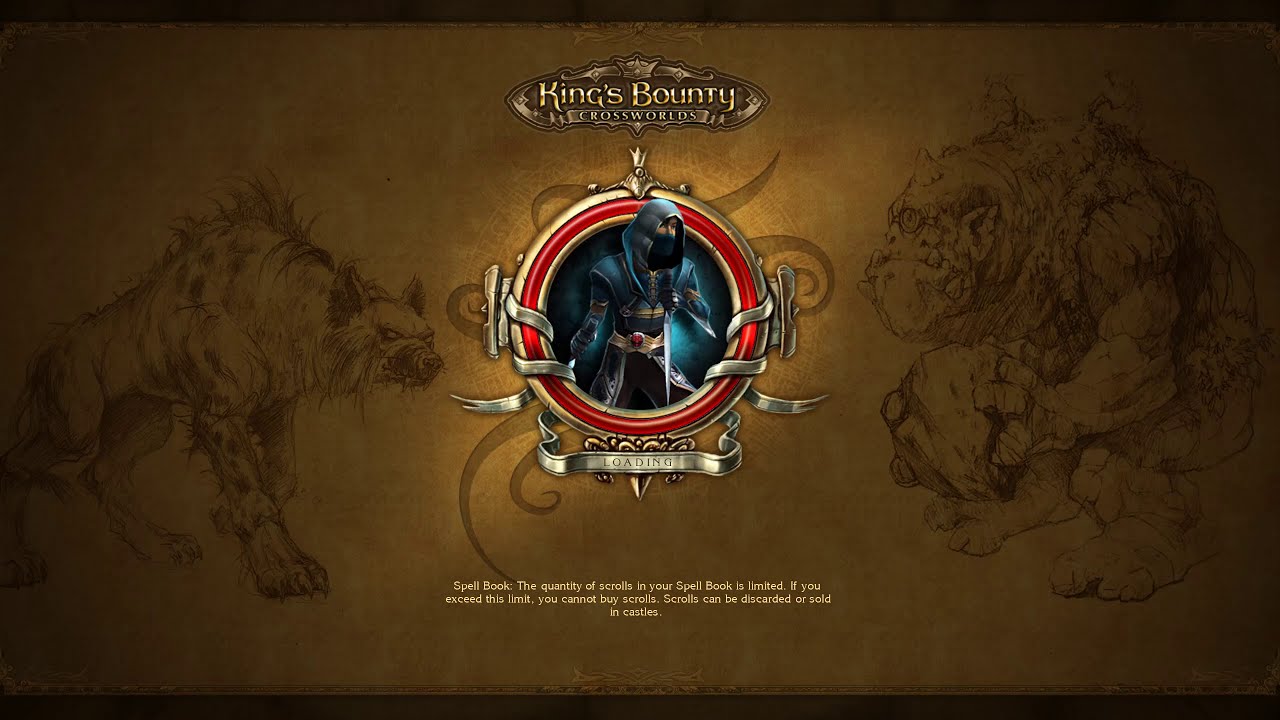This image appears to be a loading screen for the game "King's Bounty: Crossworlds." Dominating the top center is the game's title, “King’s Bounty: Crossworlds,” written in gold letters. Below the title, at the center of the image, is a red and gold circular emblem featuring a mysterious figure akin to an Assassin’s Creed character. This figure is cloaked in long robes with a hood enveloping his face in shadows. Beneath this emblem, there is an ornate silver banner that reads “Loading,” followed by a decorative scroll containing the text: "The quantity of scrolls in your spell book is limited. If you exceed this limit, you cannot buy scrolls. Scrolls can be discarded or sold in castles."

Flanking the central icon, the background is a light tan color with detailed hand-drawn illustrations of two mythical creatures. On the left side is a menacing, hyena-like beast facing right, while on the right side stands a colossal one-eyed ogre with a horn on its head. The ogre, which appears to have protruding teeth, is depicted holding a large boulder in its hands. These creatures add a formidable atmosphere to the scene, as they both seem to be watching over the circular emblem at the center.